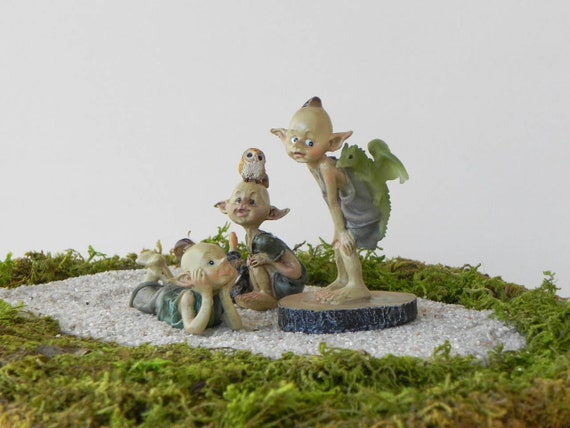The image presents a charming diorama reminiscent of Hallmark’s whimsical figurines, featuring three small garden elves or fairies set against a faded white background. The scene unfolds on a compacted stony or sandy surface, adorned with patches of fake grass or moss. Positioned on the right is a standing elf leaning forward with his hands on his knees, perched atop a slice of sawed tree trunk, with a baby dragon clinging to his back. Beside him, to the left, sits another elf with his knees drawn up to his chest, a happy smile on his face, and a baby owl comfortably nestled on his head. The third elf lies on his stomach, chin resting in his hands, gazing wistfully or pensively upwards towards the standing elf. All three elves possess pale white skin and distinctive ears that stick out like those of baby Yoda. This detailed decorative display captures a serene and imaginative moment in a miniature fantasy world.